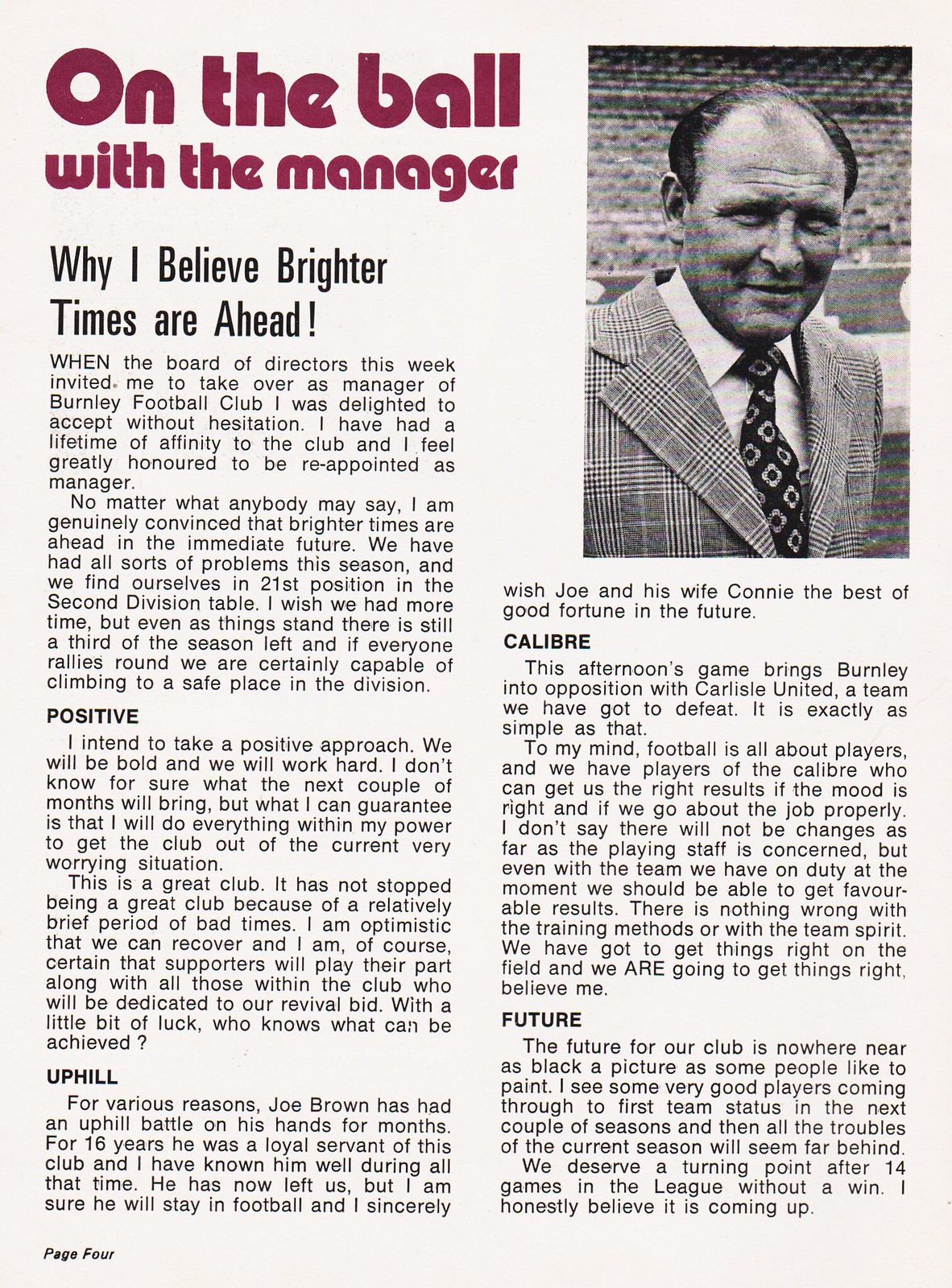The image depicts a newspaper or magazine cutout, specifically page four, which is spelled out as "F-O-U-R" in the bottom left corner. The prominent section title at the top reads "On the Ball with the Manager" in purple letters. The page features a black-and-white photograph in the upper right corner of a middle-aged man with a receding hairline and numerous wrinkles on his forehead. His eyes are shadowed, and he wears a suit with black and white stripes, paired with a black tie adorned with yellow decals, set against the backdrop of an empty stadium. 

The article is structured into multiple sections. The first section on the left at the top starts with the bold title "Why I Believe, Brighter Times Are Ahead," which is followed by two paragraphs. This section discusses the manager's new appointment at Burnley Football Club and his lifelong affinity with the club.

Below this, there is a section titled "Positive," which also contains two paragraphs. The next section, "Uphill," includes a single paragraph. Moving to the right side underneath the photograph, there is another section called "Calibre," with two paragraphs of text. The final section titled "Future" is at the bottom and consists of two more paragraphs. The article features traditional fonts resembling Helvetica.